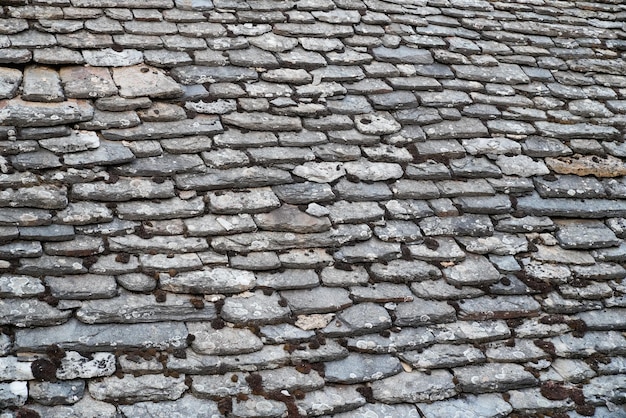The photograph depicts a close-up view of an ancient-looking stone surface, likely a cobblestone roof or path. The flat, slate-like stones are arranged in overlapping layers, creating a uniform, almost patterned appearance. Various shades of gray, with a few darker and slightly brown stones, dominate the image, emphasizing the weathered and aged nature of the material. Small weeds and patches of moss are visible between the stones, adding to the impression of significant age and exposure to the elements. The rough, chipped, and broken edges of the stones further suggest that they have endured considerable wear over time. There is no visible context beyond these stones, but the hue of the image implies an overcast, cloudy day, possibly suggesting a setting in a historical or old-world location such as the U.K. The entire frame is filled with the stone surface, highlighting the meticulous and deliberate craftsmanship behind its construction.